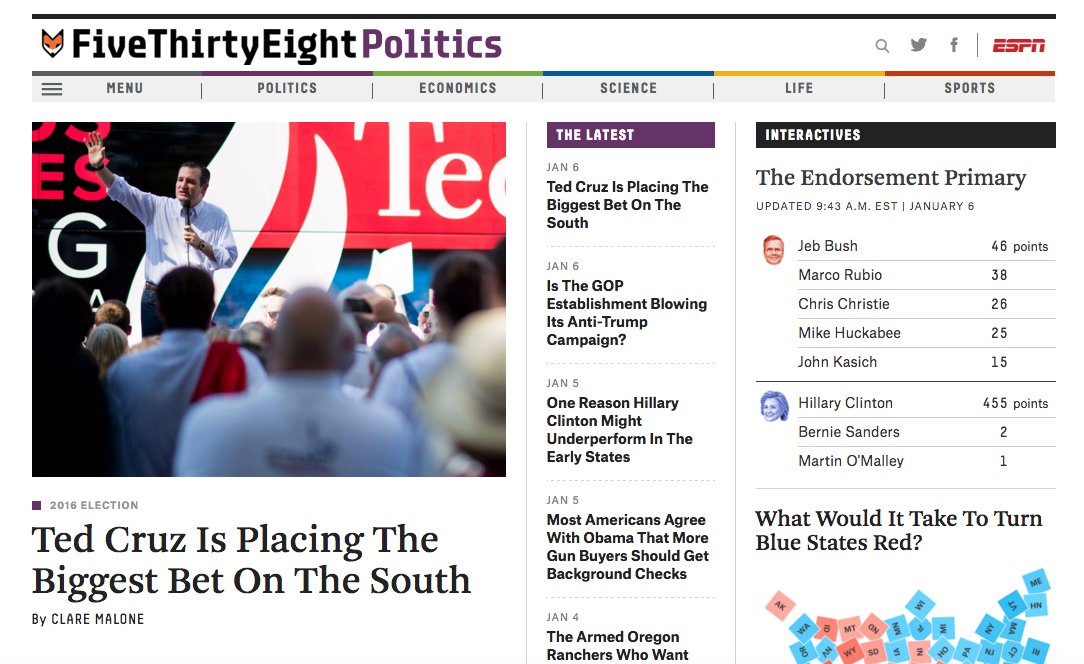Here is a detailed and cleaned-up caption for the provided image description:

---

**Politics and Endorsements During the 2016 Election**

This image captures a political analysis from the 2016 election, featured prominently on an ESPN-affiliated webpage. The site menu displays categories including Politics, Economics, Science, Life, and Sports. The headline reads, "Ted Cruz Places the Biggest Bet on the South," reflecting the intense political dynamics within the GOP and Cruz's strategic emphasis on securing southern states. The interactive graphic showcases endorsement points for Republican candidates like Chris Christie, Marco Rubio, Jeb Bush, Mike Huckabee, and John Kasich, alongside a snapshot of Democratic candidates Hillary Clinton, Bernie Sanders, and Martin O'Malley. The analysis speculates on the challenges of flipping blue states to red, hinting at the pervasive issue of misinformation. This image serves as a snapshot of the political landscape during Trump's first run for president.

---

This caption provides a coherent and detailed summary of the various elements mentioned in the original description.